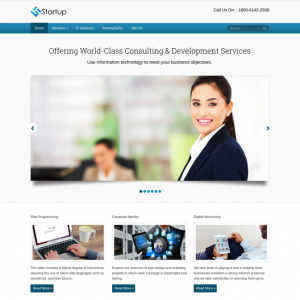This is a detailed screenshot of a website belonging to a company named Startup. At the top of the screen, there is a prominent logo accompanied by the word "Startup." On the far right, there is a small text section that reads "Call us on" followed by a phone number. Below this is a wide blue navigation bar. On the far right of this blue bar is a search option, while the left side contains other options that are too small to discern clearly.

The main title on the page reads "Offering World Class Consulting and Development Services," indicating the company's primary areas of expertise. Beneath this title, there is a smaller section of black text, but the font is too small to be readable.

Dominating the center of the page is an image featuring a woman. She is smiling warmly at the camera, dressed in a navy blazer over a white blouse. Behind her and slightly out of focus is another figure, possibly a man, who appears to be wearing a tan jacket and a white shirt; he has black hair.

Just below this large image are three smaller photographic options, likely representing various services or offerings from Startup, but the details are too small to decipher.